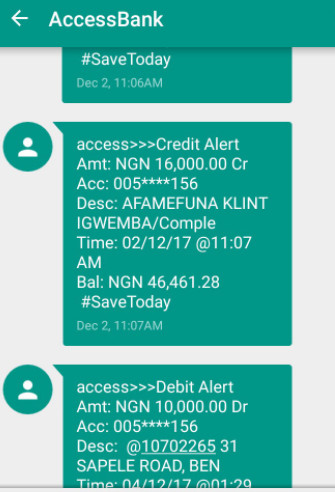**Detailed Caption:**

This image is a vertical screenshot capturing a series of messages within a mobile application. At the top of the screen, there's a teal header bar featuring white text that reads, "Access Bank" with the first "A" in "Access" and the "B" in "Bank" capitalized. Next to the text on the left side, there's a white arrow pointing to the left. A faint shadow is cast beneath the header, transitioning into the light grey background of the main screen. 

The central section of the screenshot shows teal-colored message bubbles that are rectangular and positioned in the middle of the frame. The first partially visible message bubble has white text reading, "Hashtag Save Today," with a timestamp below it in smaller, thinner white text: "December 2, 11:06 AM."

Below this bubble, another message bubble features a teal circle on the right containing a white person icon. This message reads:

- "Access >>> Credit Alert"
- "Amount: NGN 16000.00CR"
- "ACC: 0054****156"
- "DESC: AFAMEFUNACLINT"
- "IGWEMBA/COMPLE"
- "Time: 02/12/17 at 11:07 AM"
- "BAL: NGN 46461.28"
- "Hashtag Save Today"
- "December 2, 11:07 AM"

A similar message bubble follows beneath this one, with content that's cut off in the screenshot.